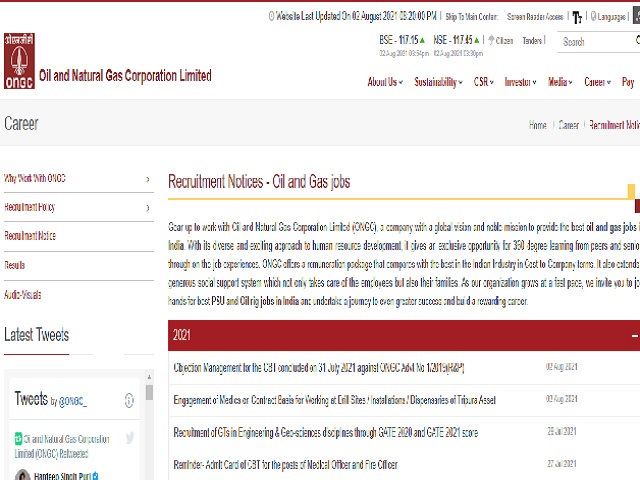Caption: 

A detailed screenshot of the Oil and Natural Gas Corporation Limited (ONGC) website. The page features text in both black and red. On the left-hand side, the ONGC logo and company name are prominently displayed. On the right-hand side of the page, there are navigational links titled "About Us," "Sustainability," "CSR," "Investor," "Media," "Career," and "Pay." The section below provides additional links related to recruitment and career opportunities, including "Recruitment," "Notices," "Oil and Gas Jobs," and a description from 2021 with an accompanying list. Beneath the "Career" section in the upper left-hand corner, options such as "Why Work with ONGC," "Recruitment Policy," and "Audio Visuals" are found.